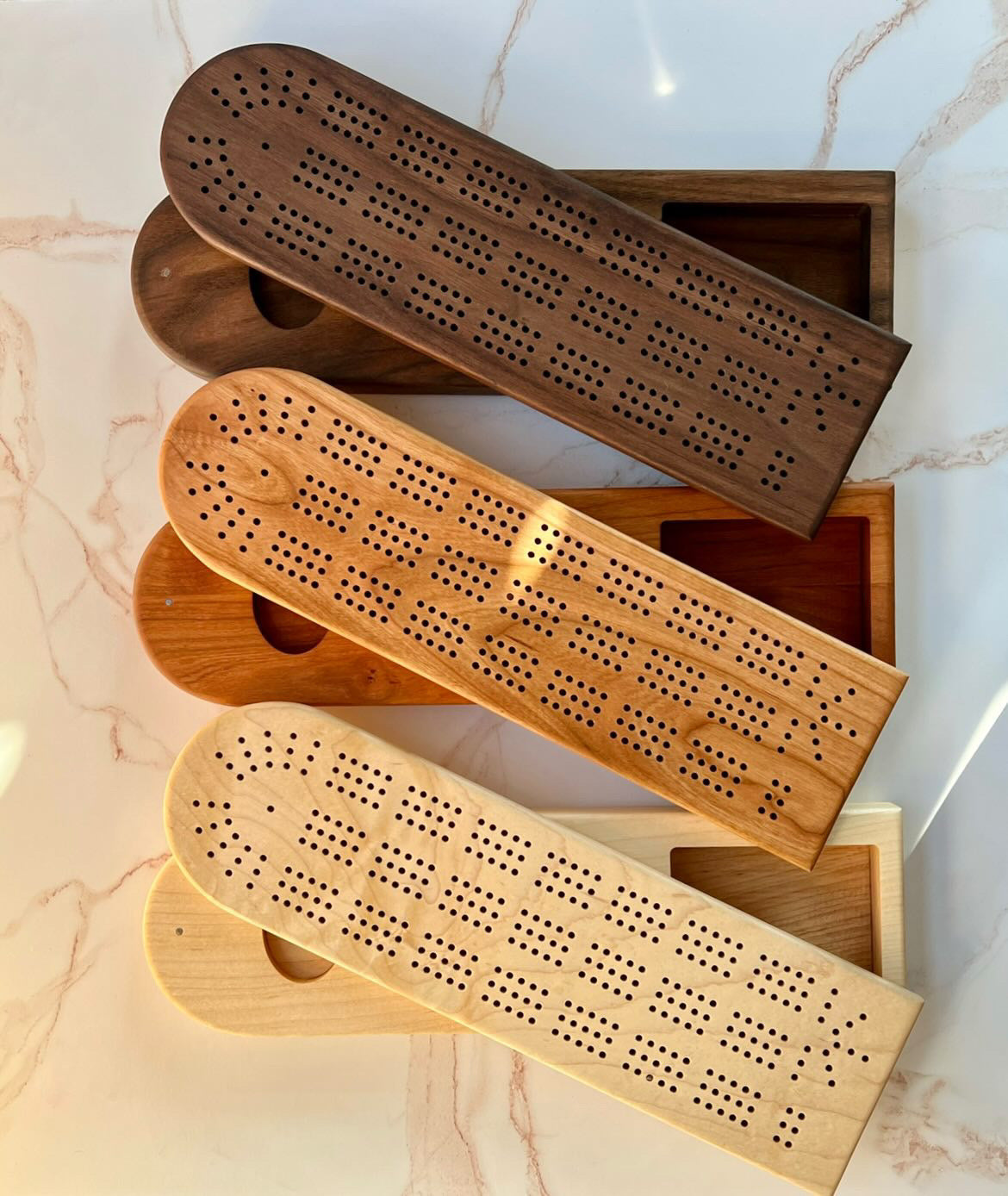The image is a vertically aligned rectangular photograph showcasing three wooden containers, each positioned within distinct horizontal segments on a white and gold marbled surface, likely a tile or counter. Each container is wider than it is tall and appears to be turned sideways, making the curved left end and flat right side visible. The containers are differentiated by color: the top one being dark brown, the middle one a medium red oak, and the bottom one a light pale wood.

Each container has a corresponding lid that lies diagonally across it. These lids share the same shape as their respective bases but are designed with vents, featuring six or seven columns of three sets of dots. The right end of each base has a cutout area revealing an internal board, with a circular hole on the left side and a larger square hole on the right side, suggesting some sort of functional design. The overall arrangement and detailed craftsmanship hint at a purposeful and intricate design, although the exact purpose of these containers remains unclear.